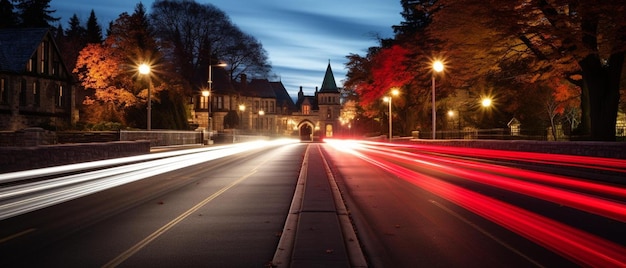The photograph captures a striking nighttime scene in what appears to be a small town or an upscale residential area with European architectural influence. Dominating the image is a central brown brick building with a distinct castle-like structure, featuring a tall, arched tower topped with a conical roof. To its left are several two- to three-story buildings with dark roofs, all adding to the old-world charm of the locale. The street, where the photo is taken from, is defined by two blacktop roads with a dark channel running through their centers. This image is particularly vivid due to the use of long exposure photography, which turns the moving car lights into mesmerizing streaks—red lights from taillights on the right and white headlights on the left—creating a science-fiction-like pattern in this historical setting. The streetlights illuminate the surrounding trees, which showcase red and orange leaves, indicative of the fall season. The skyline is somewhat cloudy, with a moody evening ambiance, amplifying the photograph's enchanting and dynamic qualities.